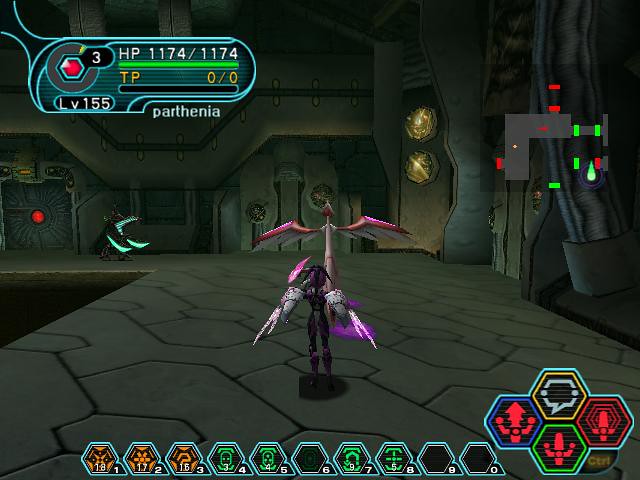In this captivating screenshot from a video game, the main character is prominently centered on the screen, adorned in dark purple attire. Their ensemble includes distinct white gloves or gauntlets that feature pink accents. Engaged in a tense battle, the protagonist faces off against a small dragon-like enemy, colored in shades of white and pink.

In the upper right corner, a mini-map provides a strategic overview of the area, depicted as a gray L-shaped block. The map includes red lines indicating locked doors and green lines representing accessible paths. The top left corner displays the character's health bar, reading "1174 out of 1174" with a corresponding green bar, along with statistics such as "TP: 0 of 0" and "Level: 155." Also present is a red gem icon with the number "3" adjacent to it, and the name 'Parthenia' is clearly printed in white text.

The setting features a brown and gray floor with a geometric pattern, suggesting a high-tech environment that resembles a spaceship or spacecraft, complete with airlocks and other space-specific design elements.